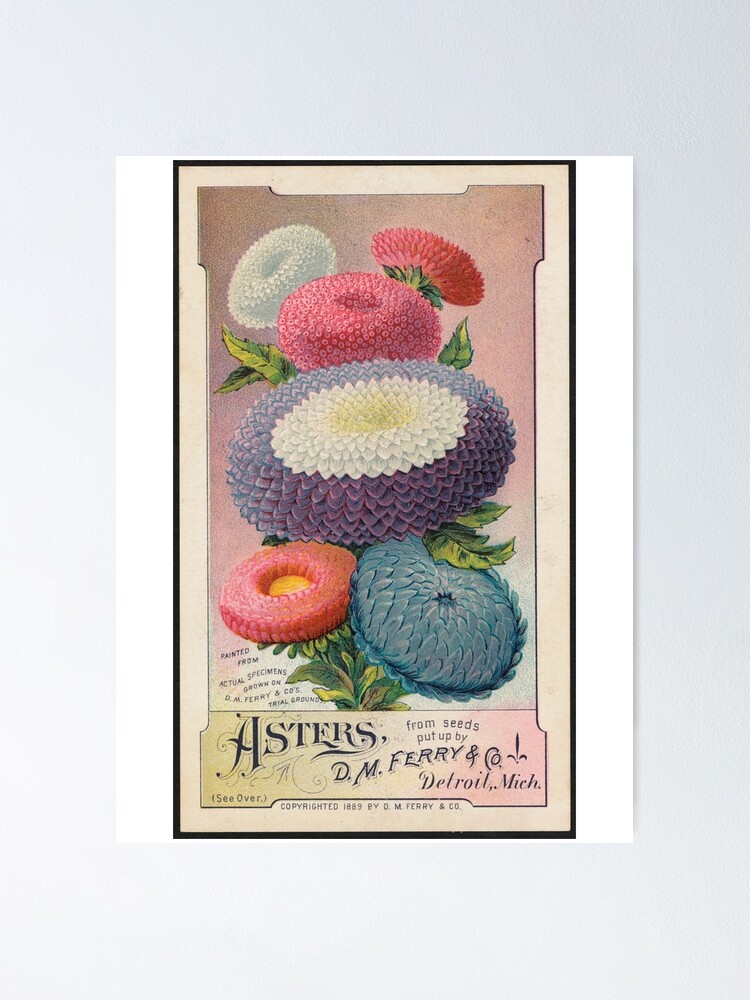This detailed and vibrant advertisement poster is for "Aster's from Seeds Put Up By D.M. Ferry and Company, Detroit, Michigan." Set against a decorative, multi-layered background, the poster features several uniquely colored flowers arranged artistically. The outer edges are framed with white borders, followed by a black border, and then a pink backdrop. The central image showcases six distinctive flowers, each round and donut-shaped, with varied color schemes. 

At the top left, there is a bluish flower facing up and to the left. Below it lies a pinkish flower with a dark spot in the center and green leaves extending to the sides. Adjacent to these is another flower seen from behind, displaying a pink back with a hint of green. In the center of the poster, a larger purple flower with a white center stands out, accompanied by leaves on its lower right. Below this are a pink and yellow flower facing upward and a slightly larger all-blue flower. This floral arrangement is surrounded by numerous green leaves. 

At the poster's bottom, a banner spreads across the green leaves, containing black lettering with the advertisement's text. Despite the ornate visual presentation, the background maintains a clean and soft grayish-white shade, ensuring that all elements stand out vividly.